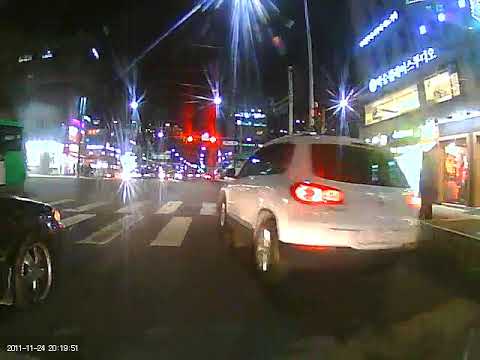This is a blurry nighttime photograph, likely dash cam footage, capturing a bustling city street. The focal point is a white Volkswagen SUV driving down the road, accompanied by a black car to its left, with its front wheel just visible. The image is characterized by bright, blurred lights from street lamps, traffic signals, and possibly reflections from nearby skyscrapers, giving the scene a star-like appearance. The street is marked by white crosswalk stripes, and various signs with what appear to be Asian characters, possibly Korean or Japanese, are discernible. A red light streak, potentially from a traffic signal, adds to the visual confusion. A time stamp in the bottom left corner indicates that the photo was taken on 2011-11-24 at 20:19:51 (military time), grounding this dynamic urban scene in a specific historical context.